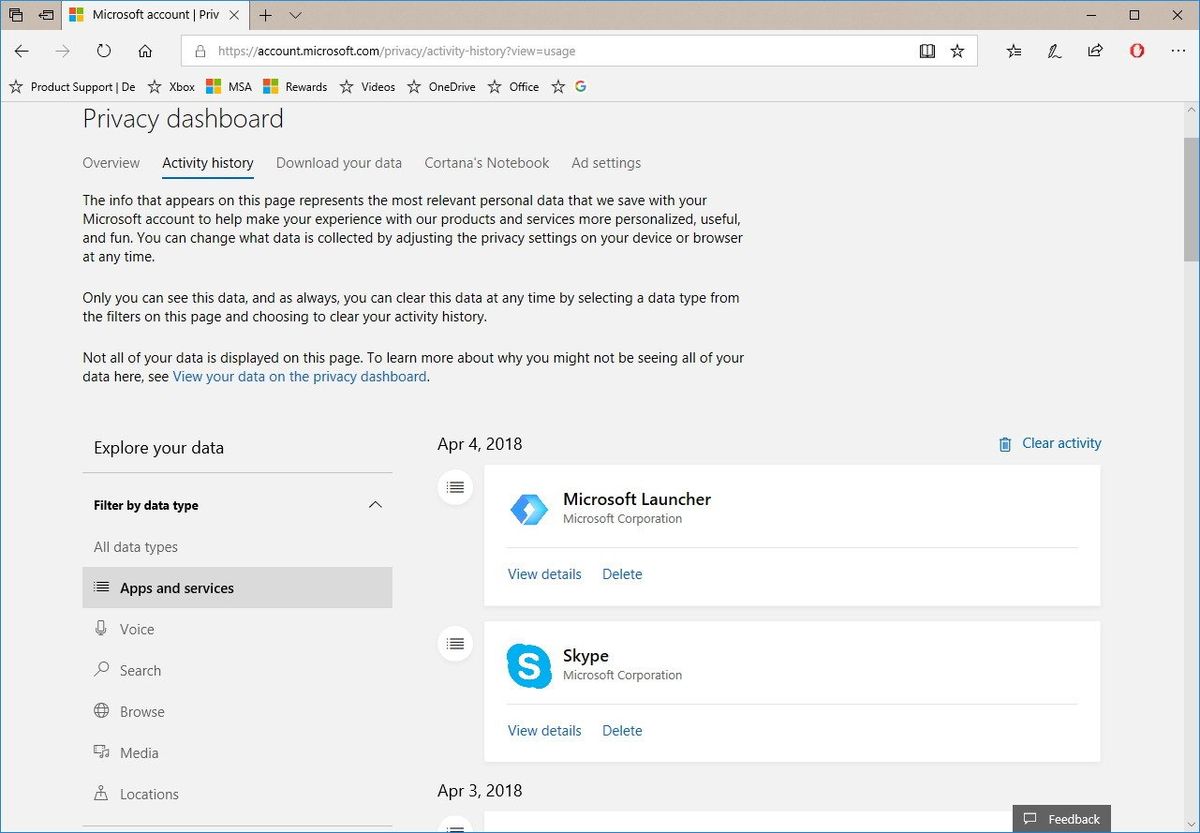The image depicts a Microsoft account webpage, specifically the "Privacy Dashboard" located at account.microsoft.com. The top of the page prominently displays the title "Privacy Dashboard" against a clean, white background. Beneath this header, several navigation buttons are visible, labeled "Activity History," "Download Your Data," "Cortana's Notebook," and "Ad Settings."

Further down, a detailed explanatory message is presented. It informs the user that the displayed information represents the most pertinent personal data associated with their Microsoft account. This data is used to enhance the personalization, utility, and enjoyment of Microsoft's products and services. Users are informed that they can modify the data collection by adjusting their device or browser's privacy settings at any time. Additionally, the message assures that the data is visible only to the user and can be cleared whenever desired by selecting a data type from the provided filters and opting to clear the activity history.

The note also clarifies that not all data might be displayed on the page and provides a hyperlink for users to click to learn more about the potential reasons for this absence. Finally, there is a clickable area labeled "View Your Data on the Privacy Dashboard," inviting users to explore their stored information in more detail.